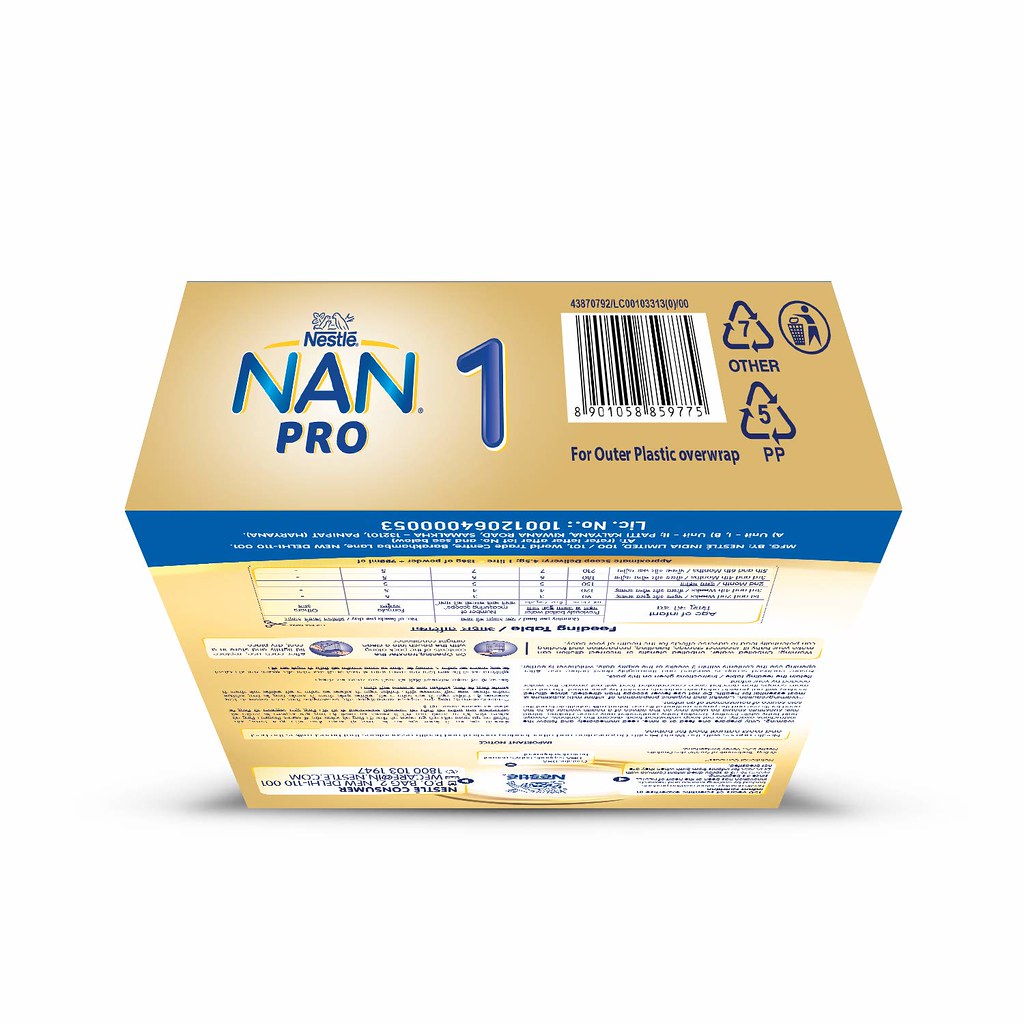The image depicts an upside-down cardboard packaging for the product "NAN Pro 1." At the top of the box (which is actually the bottom due to its orientation), there is a blue strip. Above the main product name, there is a yellow stripe that features the Nestle logo in the center. Just to the right of the "NAN 1" label, there is a barcode accompanied by text stating "For outer plastic overwrap." Below the barcode, there are two or three recycling triangles indicating recyclability. In the top right corner (bottom left due to the inversion), there is an icon of someone throwing something into a trash can, circled for emphasis. The text on the back of the box, including the nutrition label and serving size information, is also upside down, making it clear that the entire box is positioned incorrectly.